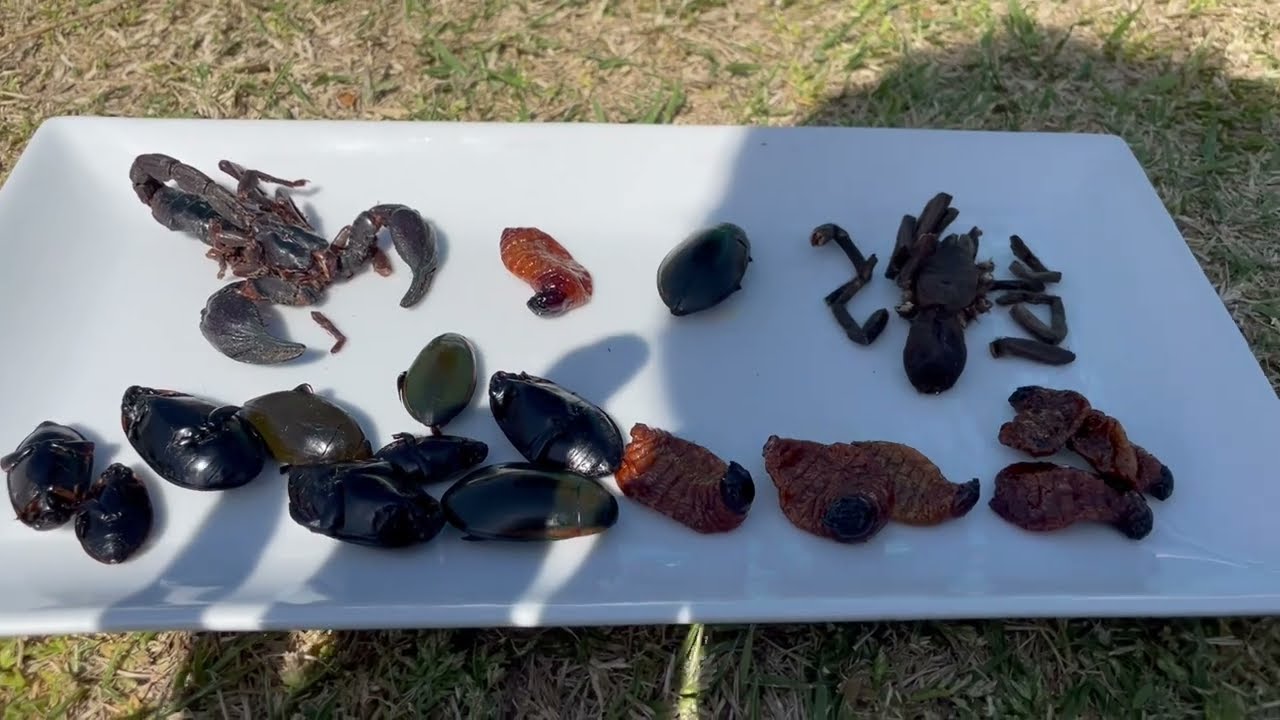The photograph showcases a white rectangular ceramic tray placed on yellowing grass and surrounded by desert-like foliage. The tray displays an assortment of seafood remnants and various large insects, including crabs, mollusks, bugs, larvae, and even a scorpion positioned at the top-left corner. The seafood and bugs, with hues ranging from black and dark greenish-gray to orange, appear sorted by color and shape. The arrangement suggests either an entomological collection or preparation for cuisine. The items on the tray, numbering around 18 to 20, seem to be in mixed conditions, with some completely intact while others are fragmented. The daylight setting enhances the vivid details of the unusual assortment.